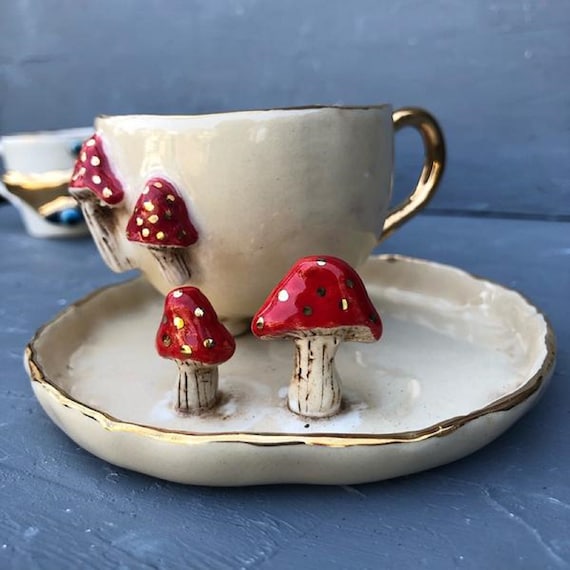A detailed photograph showcases a whimsical handmade teacup and saucer set, positioned centrally on a dark grey, painted wooden table. The table's grain pattern is visible beneath the brush strokes of thick grey paint. The background wall also bears the same dark grey hue, creating a cohesive, moody atmosphere. 

To the left, slightly out of focus, sits another cup or mug adorned with striking gold and blue details. 

The teacup and saucer in the center are the centerpiece of this image. The teacup features charming design elements: a red-capped toadstool with white (occasionally gold-reflective) spots on the left side, and a handle positioned to the right. A lustrous gold rim adorns the top edge of the teacup, adding an elegant touch. 

The accompanying saucer, appearing much like an inverted flat mushroom with a pronounced lip, also boasts a gold-edged detail. The handmade nature of the piece is evident in its rough, scalloped edges and non-uniform shape. Additionally, two red-capped, white (or potentially gold) spotted toadstools stand attached to the saucer, enhancing the whimsical and enchanting aesthetic of the set.